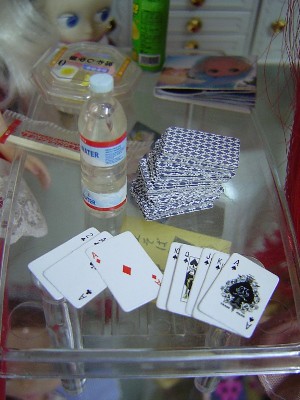The image is grainy and slightly out of focus, capturing a cluttered and intriguing scene. At the very top, there is a face with striking blue eyes gazing towards a light source, framed by almost white, blonde hair. On the right-hand side of the image, there is a unique green and yellow patterned cat, positioned near what seems to be a nutrition label in black text.

Behind this, a dresser with three visible drawers and distinctive yellow handles occupies the background. Just to the far right, strands of pink hair dangle from above, adding an unusual splash of color. Next to this, a book rests on a table, its cover displaying the face of a doll. 

On the left-hand side of the image, a clear plastic container holds an unknown food item, with Eastern text adorning its surface. Nearby, chopsticks are neatly placed inside another plastic container. Also visible in this area is a water bottle, sealed with a light blue label accented by a red strip at the top, completely filled to the brim.

At the bottom of the scene, a stack of playing cards featuring a blue back with a diamond pattern is partially buried. A fanned array of cards indicates a sequence starting with two of spades, then ace of spades, followed by ace of diamonds, king of spades, queen of spades, jack of spades, another king of spades, and finally, another ace of spades.